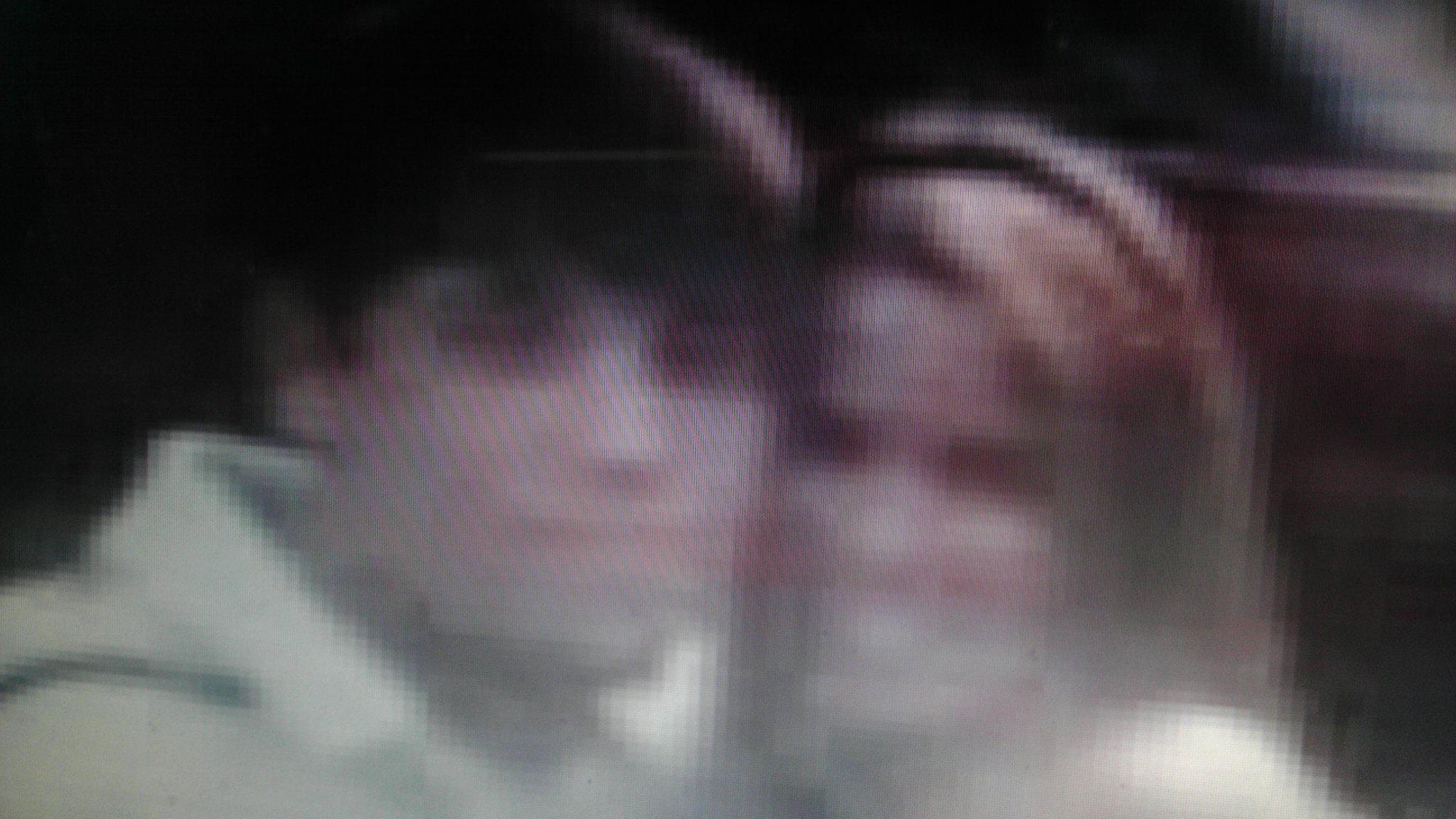This is a photograph, likely from the 1990s, depicting either siblings or a couple seated closely together. The image, which is quite blurry and marred by black spots, suggests considerable age and wear. It features a Caucasian male and female, with the woman smiling warmly while the man maintains a neutral expression. The woman's blonde hair is adorned with a headband, and she appears content and cheerful. The man, clad in a hoodie or sweater, contrasts her expression with a more reserved demeanor. The colors in the photo are muted, contributing to its nostalgic and worn appearance.